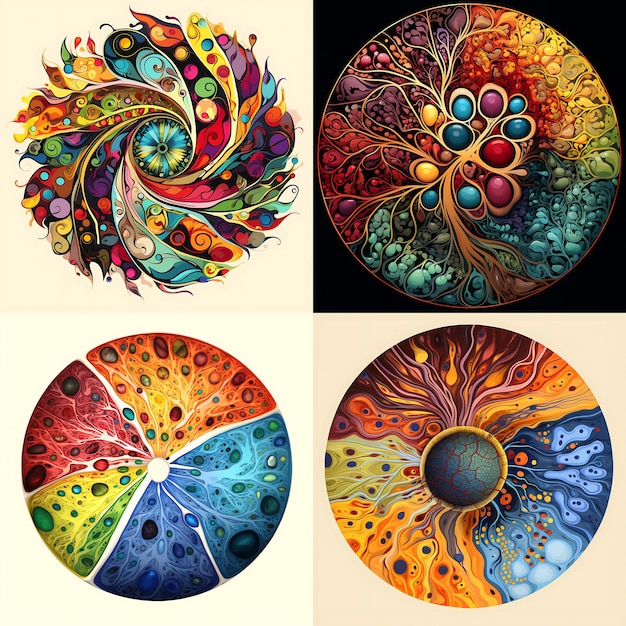This image showcases four distinctly psychedelic circular patterns, arranged in a 2x2 grid, each brimming with vibrant colors and intricate designs. The top left circle features a mesmerizing swirl that converges to a metallic aqua and lime green center, reminiscent of a black hole pulling in fragmented hues of blues, reds, and greens against an off-white parchment-like background. Moving to the top right, a black background highlights a formation resembling eggs or plant roots, with maroons, reds, yellows, lime greens, and bright blues intricately woven together in an hypnotic dance. The bottom left circle presents a mosaic of oil-like blobs separated into pie-piece segments, each infused with vibrant shades of aqua, purple, lime green, yellow, bright red, and orange, set against an off-white backdrop. Finally, the bottom right circle evokes the imagery of a planet or an eyeball with paisley prints and swirling veins in orange, surrounded by a psychedelic mix of colors, also on an off-white background. Each design is a kaleidoscope of 'hippie' colors and abstract shapes, interweaving dots, swirls, and patterns, creating a captivating visual array.